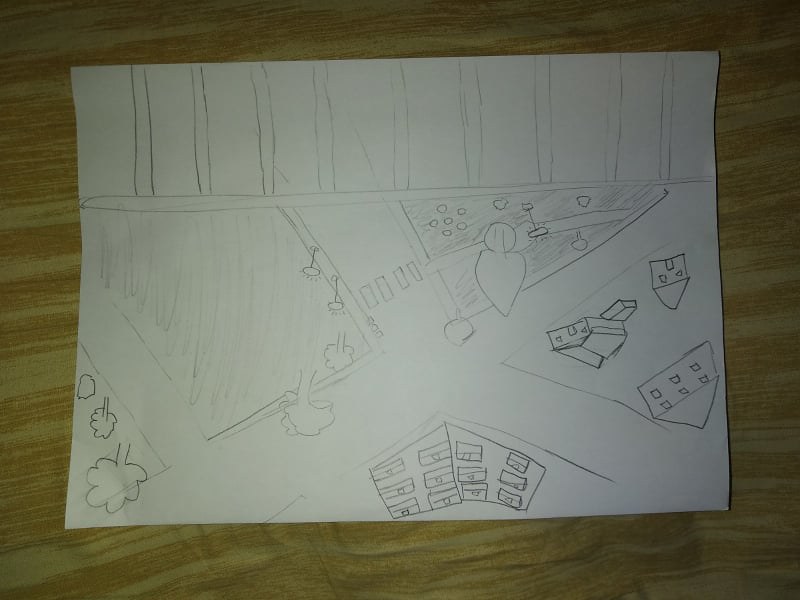This intricate pencil drawing, laid out like an aerial view of a city street map, rests on a dark to medium brown table adorned with wavy white stripes that create a visual contrast to the pristine white paper. The drawing appears almost inverted, adding a unique perspective.

Starting from the upper edge, dual parallel lines run downward and then across, creating a grid-like structure. Just left of the center, a prominent street emerges. Flanked by sidewalks on both sides, this street is detailed with a couple of streetlights on the left side. Adjacent to the street, a block features a park, identifiable by a crosswalk leading to it, a single tree, a stoplight, a few bushes, and grassy areas. The sidewalk meanders beneath the tree, wrapping around the light, and connecting back to the road.

Diagonally cutting across the paper from the bottom left to the upper right is a significant road. The field that the top road feeds into is an open grassy space with scattered trees. To the left edge, another road exits, bordered by a small block with more trees. Dominating the bottom section of the drawing is a large block housing a conspicuous three-story building, indicated by twelve windows arranged in three rows of four and a marked corner line.

Entering the fifth block, the drawing reveals additional residential elements, including a couple of houses, completing the detailed urban landscape.